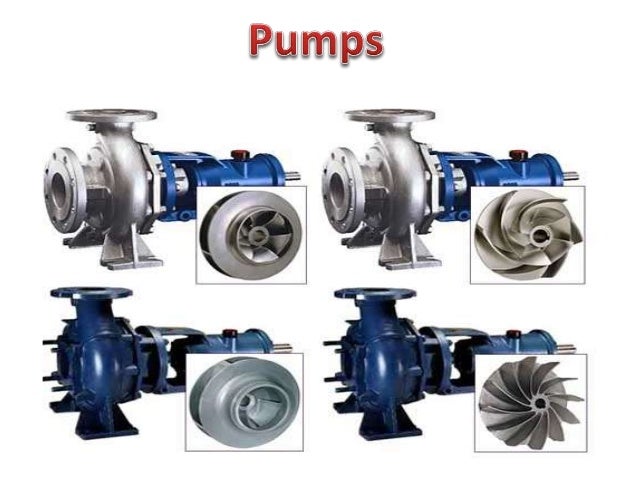The image displays four displacement pumps in a grid arrangement, with two pumps on the top row and two on the bottom row. Each pump features a different impeller design. At the top of the image, the word "PUMPS" appears in bold red font with a white outline and shadows.

Starting in the upper left, the first pump's body is a combination of silver and blue. An inset box shows the impeller, revealing a smaller circle with several fins inside, resembling a mini fan blade with six blades. The second pump, positioned in the upper right, also has a silver and blue body. Its impeller features larger fins extending to the edge of the blade, with a more cylindrical appearance and a center shifted slightly to the right.

In the bottom row, the pump on the left is entirely blue. The inset image of its impeller shows a smaller circle with one or two very thin blades inside. The final pump on the bottom right also has an all-blue body. Its impeller design comprises many blades forming a twisted star pattern, with the blades reaching out to the edge.

Each pump is accompanied by a white box with gray lines showcasing the impeller's view. The descriptive elements emphasize the color scheme and unique impeller designs, providing a detailed comparison of the four pumps.